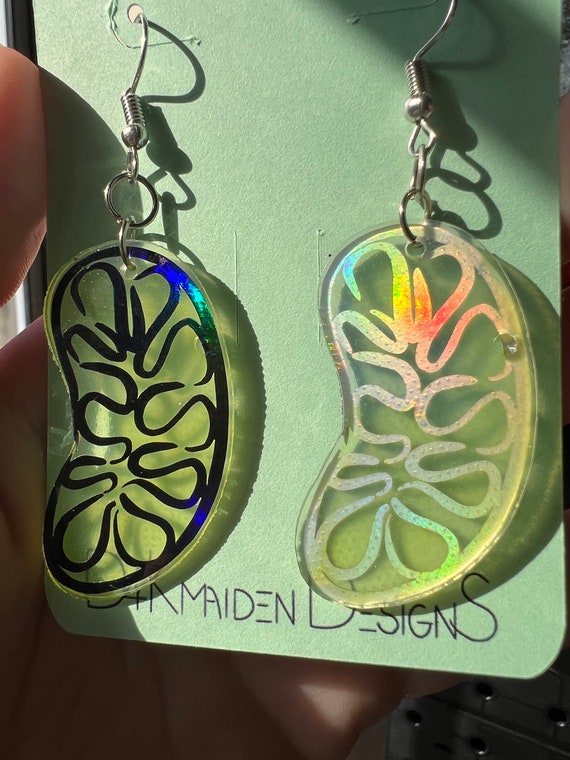The image is a vertically-aligned, close-up product photograph showcasing a pair of hook-style, dangling earrings. The earrings are displayed on a light green cardstock backing, with small holes at the top for hanging. At the bottom of the cardstock, in black, all-caps text, it reads "Dan Maiden Designs." Each earring features silver hooks on top, connected to a small circle and ring that attach to the actual earrings. The earrings themselves are flat, acrylic, bean-shaped with various black, swirled squiggle marks and a border around the edges. The right earring displays a colorful design of yellow, blue, and pink, while the left one has a monochromatic black design. The cardstock and earrings are being held by someone's left hand, visible on the far left side of the image.